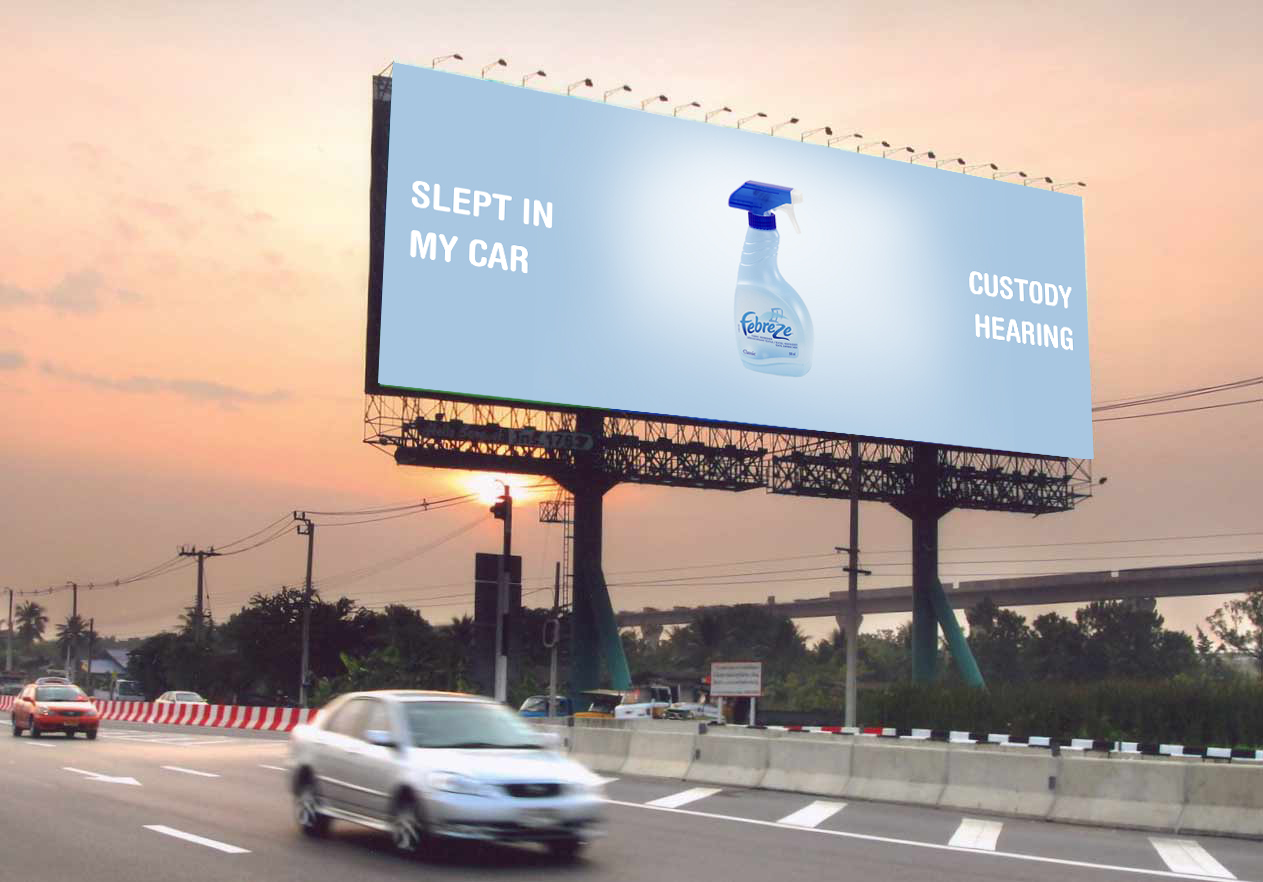An evocative sepia-toned photograph captures a bustling highway at sunset, featuring a prominent billboard that dominates the scene. The billboard, centered diagonally from the 3 o'clock to the 11 o'clock position, advertises Febreze fabric spray with a striking image of a white bottle adorned with a dark blue spray nozzle. The bottle, highlighted by a lighter gray area in the center, prominently displays the blue "Febreze" lettering. Flanking the bottle, bold white text reads "Slept in My Car" on the left and "Custody Hearing" on the right. Above the billboard, a row of about 12 to 15 small lights sits ready to provide nighttime illumination. Below the advertisement, concrete barriers with sections painted black and white divide the highway, which is under construction and marked by red and white plastic barricades. On the highway, a blurry silver sedan speeds to the right while a red car in sharp focus lingers behind. Telephone poles with connecting wires stand along the roadside, and the entire scene unfolds against a backdrop of pinkish-orange hues from the setting sun, casting a peaceful glow over distant trees.